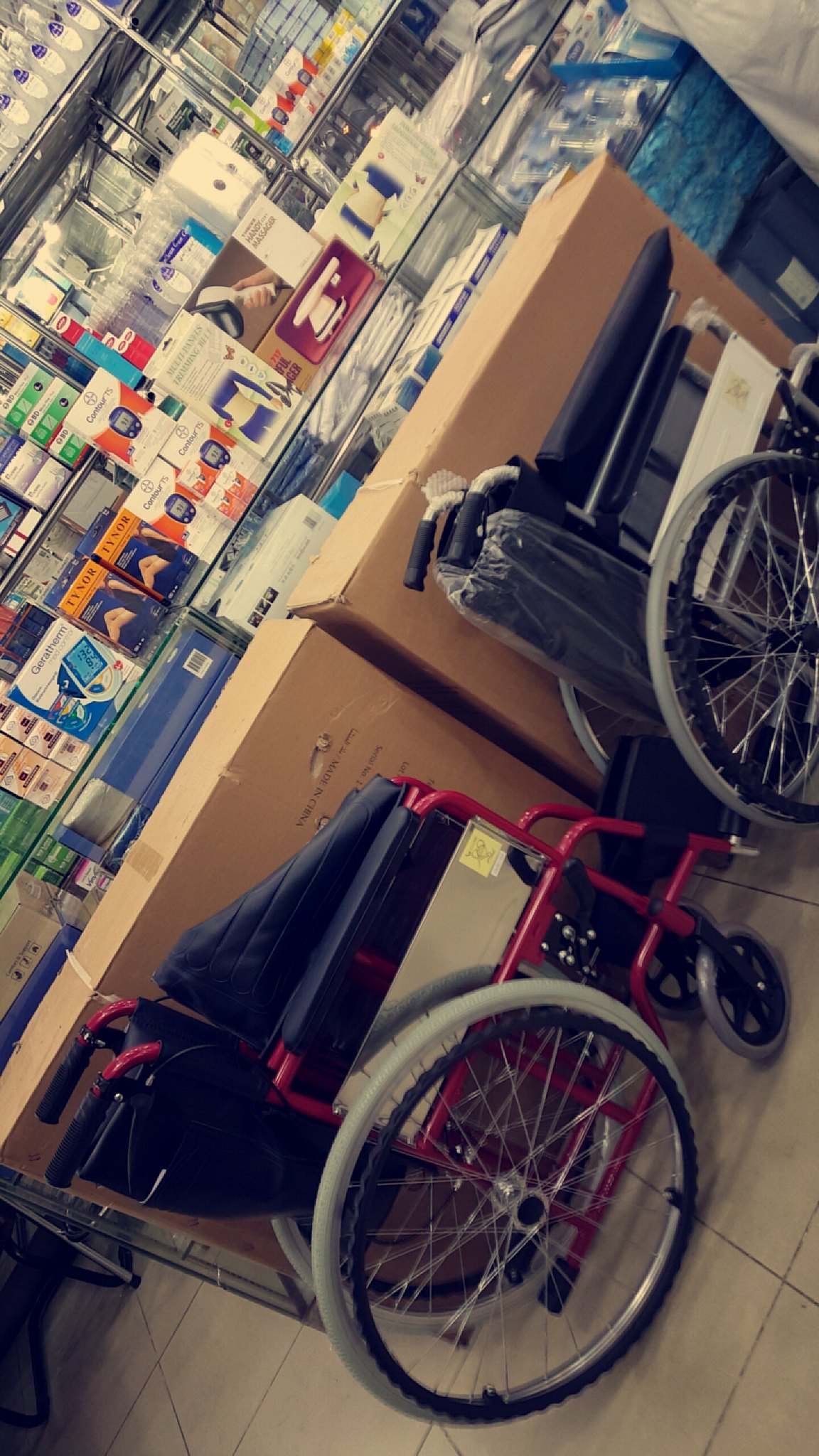The image captures the interior of a versatile store, potentially a medical supply or drugstore, with an off-white tiled floor. In the foreground, two folded wheelchairs are prominently displayed, each featuring white wheels with black rims. One wheelchair has a red frame and a blue seat, while the other is black. Behind them lie two brown boxes, presumably the packaging for the wheelchairs. The background reveals a cluttered glass counter housing various electronics and medical items. On the walls, a variety of products are visible, including workout equipment, electronics, sanitizer, and medical supplies like bed sheets and a blood pressure monitor in blue and white packaging. The photograph is taken at a slight angle, making the arrangement of items appear somewhat askew.